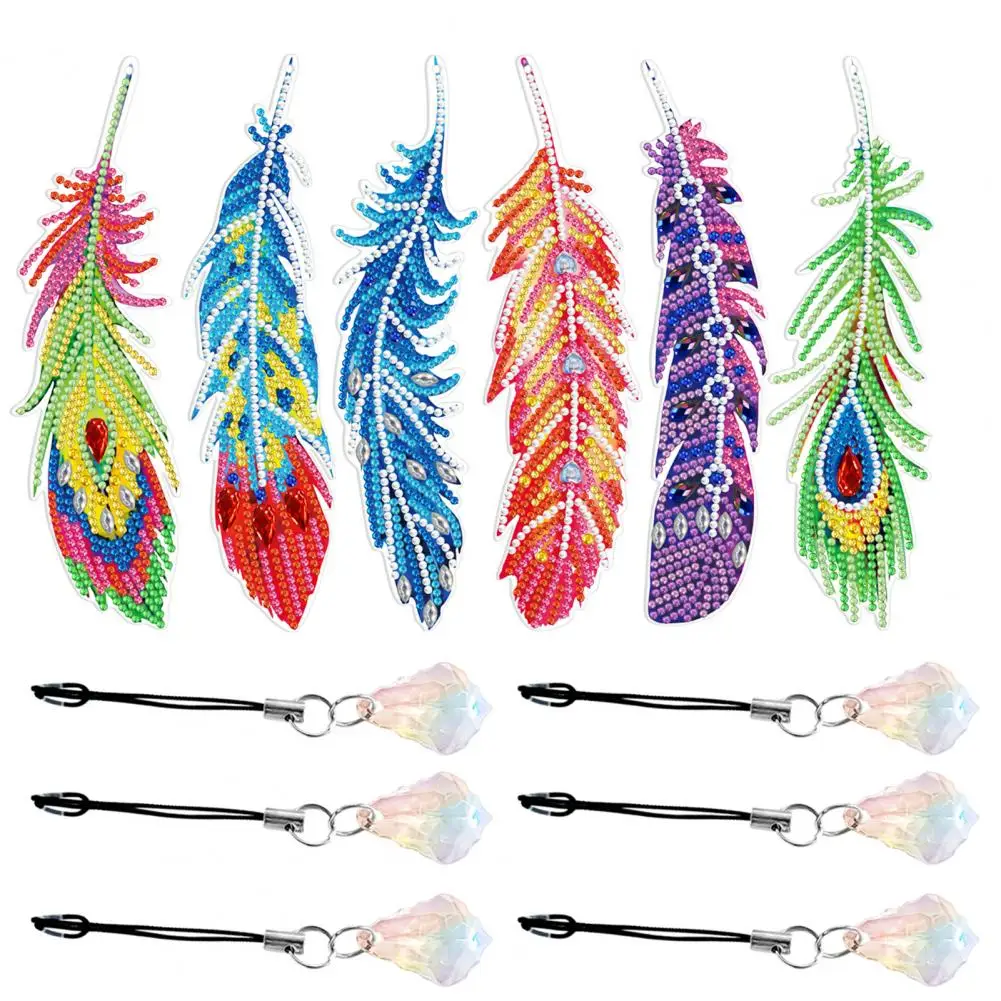The image features six intricately designed keychains or keepsakes that are arranged in a row. Each keychain displays a vibrant feather made from tiny, colorful beads. The feathers are oriented downwards with stems at the top, which are either green or white. The first feather displays hues of red, pink, yellow, and green, with colors blending as they taper down to a tip. The second feather features an array of blues, yellows, reds, and oranges. The third feather is a mix of white and various shades of blue. The fourth one combines shades of pink, orange, and white. The fifth feather includes a distinctive circular design in the center, composed of a blue core with a white outer ring, and the rest of the feather is decorated with blue, purple, pink, and white beads. The final feather begins with green wisps, followed by a blue teardrop with a red center, transitioning into yellow and green again.

Underneath these beaded feathers are string or leather cords laid horizontally from left to right. At the end of each cord, there is a silver metal clasp with two metal rings attached to it, and further attached is a multifaceted, pale-colored crystal stone that showcases shades of pink, white, blue, and purple. Each keychain thus combines both the intricate beadwork of the feathers and the elegant simplicity of the crystal stones, creating decorative items that look both colorful and artistic. The background of the image is white, enhancing the vivid colors of the displayed items.